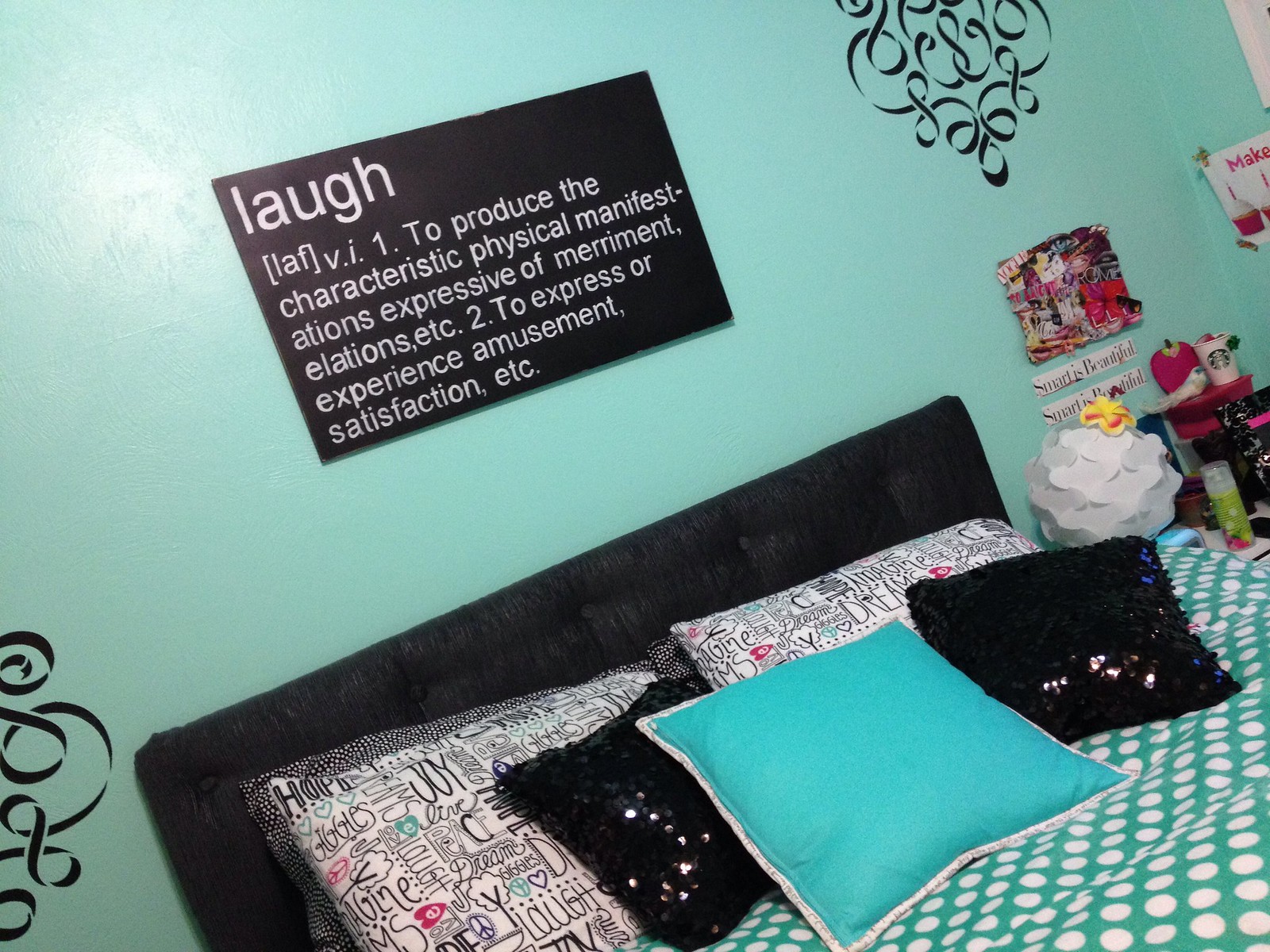This photograph captures a cozy and chic bedroom setting with a prominent sky blue, or light teal, wall as the backdrop. The focal point is the stylishly designed bed, accented by a black padded headboard. Adorning the bed are five distinct pillows: two white pillows featuring a busy design with black text and some pink elements, two smaller black pillows adorned with sequins, and a vibrant sky blue pillow with a white border. The bedspread matches the pillow, being sky blue with white polka dots.

Above the headboard, a large black sign with white text prominently displays the definition of the word "laugh," detailing its physical manifestations and emotional experiences. The photograph, presumably taken with the camera tilted to the left, adds a unique perspective, aligning everything in the image at a slight angle.

To the right, a white decorative lamp stands on a desk, accompanied by a Starbucks coffee cup and an assortment of handcrafted collages affixed to the wall, enhancing the personal and creative ambiance of the room.